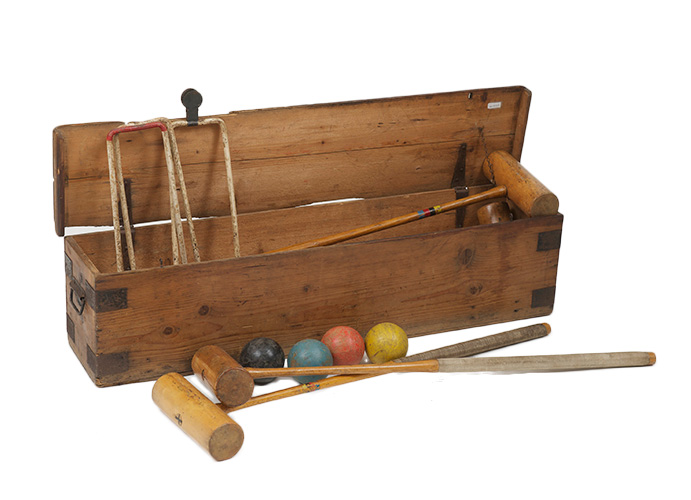This image depicts a vintage croquet set contained in a long, rectangular, light brown wooden box. The box's lid is open, revealing its contents, which include a mallet and several white metal arches or gates used in the game. The box is reinforced at the corners with dark brown metallic brackets and features handles mounted on both sides. There is also a piece of white paper taped in the upper right corner of the box. 

In front of the box, two croquet mallets rest with their hammer ends pointing to the right. The handles of these mallets are worn, showing some chips and cracks, indicating extensive use over time. Behind the mallets are four brightly colored balls: one black, one blue, one red, and one yellow. All elements of the kit, including the balls and the box, appear weathered and aged, adding to the vintage aesthetic of the set.

In addition, the box has two rectangular pieces on the left side that extend to the top, with a black circular flap protruding from one of them. The background of the image is completely white, highlighting the rustic charm and historical feel of the croquet set.